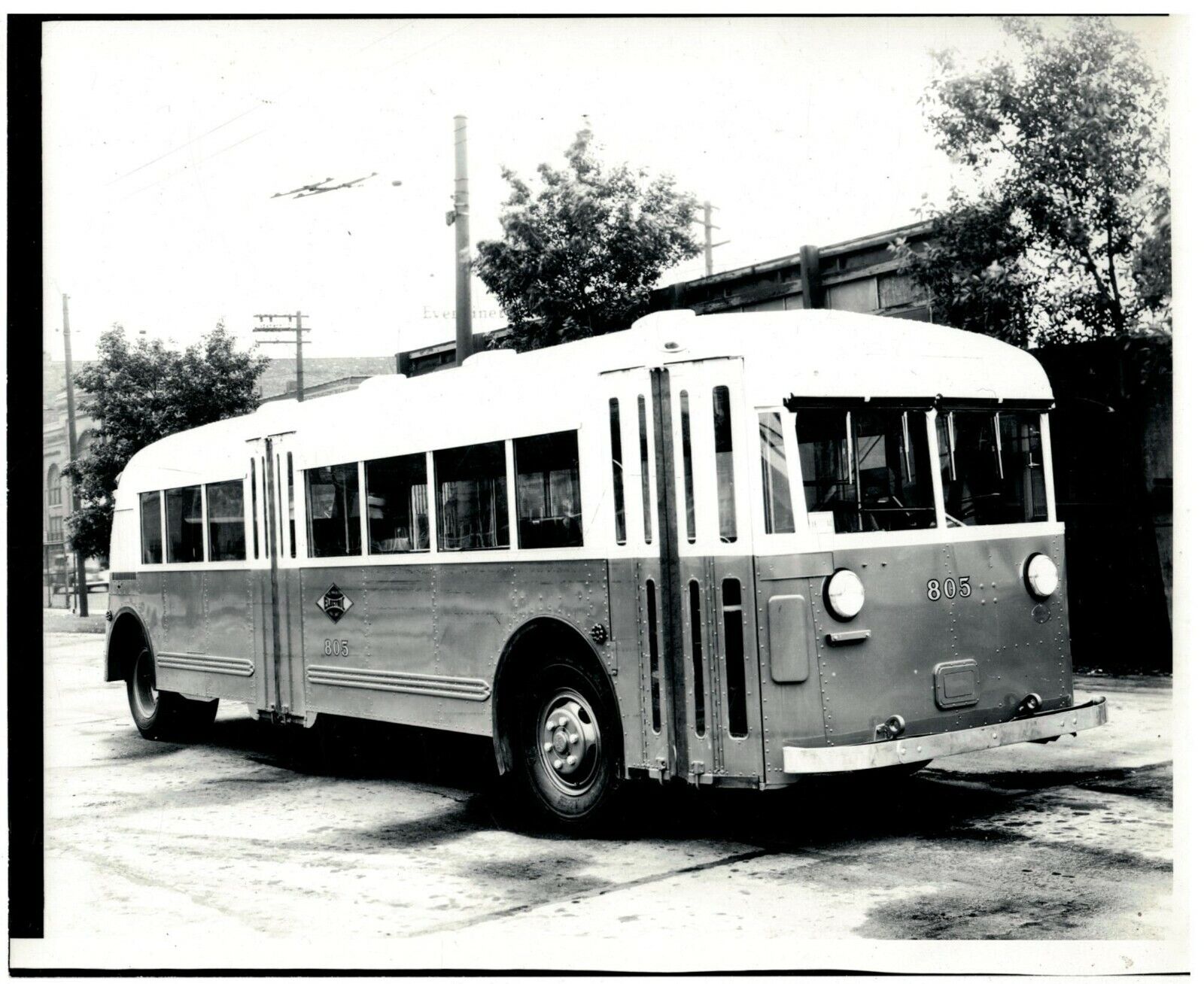This detailed black and white photograph depicts an old bus numbered 805, prominently positioned facing right and slightly towards the camera on an asphalt street. The bus, with a dark lower half and a white upper half, features a distinct diamond-shaped logo on its side and two circular headlights on the front. Visible are numerous windows and a door on its left side, near the curb. Surrounding the bus is a sidewalk, with telephone poles and power lines stretching along the street. The backdrop includes a series of trees, a few buildings, and a tall fence on the right. The photo was likely taken during the day under a white sky, with hills or mountains faintly visible to the left and above. The scene is devoid of any people or other vehicles, adding to the focus on the vintage bus.